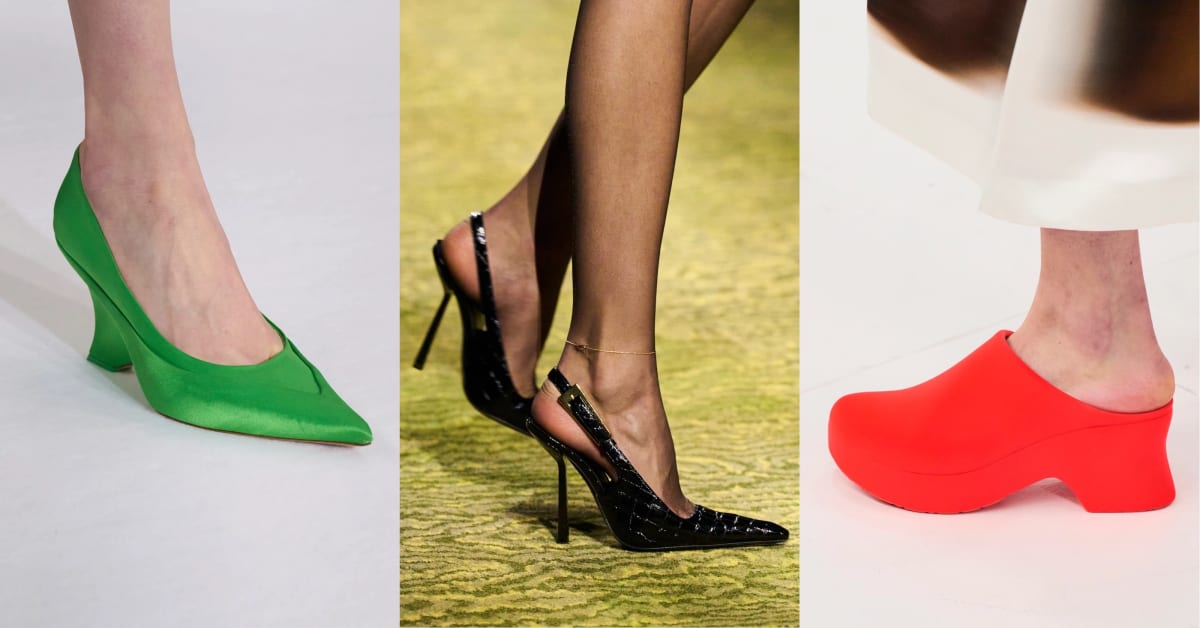The image features a series of three distinct photos showcasing different styles of women's footwear against varying backgrounds. On the left, there is a single foot adorned in a sleek, emerald green high-heeled pump with a pointed toe, likely made of satin, set against a white background. The center photo displays two feet wearing glossy black stiletto slingback pumps, possibly fashioned from crocodile skin, with an anklet adorning the right foot; both feet rest on a green and brown carpet, with one foot slightly lifted. Lastly, the right image highlights a foot in a striking neon red, backless clog with block heels and a rounded front, emerging from beneath a white skirt with a brown hem, also on a grey background. This trio of images captures a variety of footwear styles, materials, and colors.